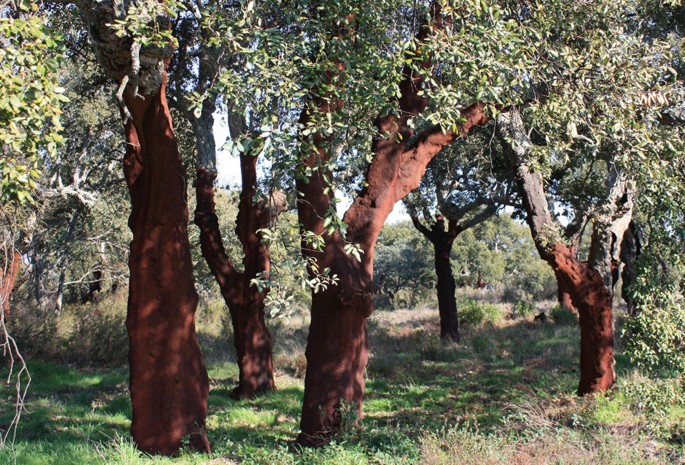The photograph captures a serene forest bathed in bright sunlight, creating peculiar shadows and an overall luminous atmosphere. The forest, which isn’t overly dense, features open spaces allowing ample sunlight to flood the area. In the foreground, there are prominent trees with thick trunks; the most striking feature of these trees is their unusual coloration—a matte, lava-like red surface that appears almost painted, contrasted by the natural grayish bark seen on higher branches. The forest floor is covered with lush green grass interspersed with some brown patches. The background reveals a blue sky with white clouds hovering above a canopy of green foliage. There are no human elements, paths, or signs in sight, emphasizing the untouched and natural beauty of the scene.